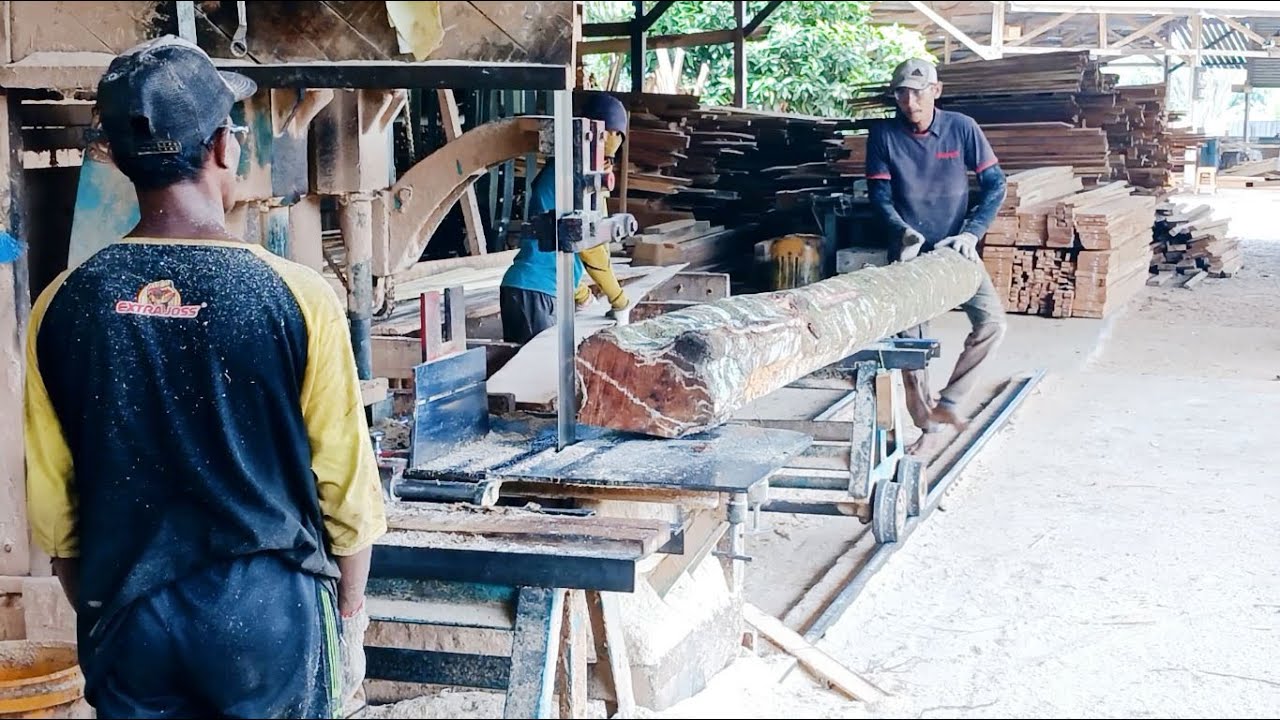In the bustling lumber yard, surrounded by stacks of processed wooden boards, three workers are hard at work on a large tree branch, preparing it for further processing. In the foreground, two men clad in blue hats and blue pants, both wearing gray gloves, are intently focused on their task. One man, in a blue and yellow shirt and glasses, stands ready with a large silver-and-black machine equipped with a white handle, positioned on a blue table dusted with sawdust. His colleague, dressed in a blue shirt with red stripes, khaki pants, and boots, assists him. A third man can be glimpsed in the distance, wearing a blue shirt and white pants, barefoot despite the harsh environment. Numerous wooden boards, both processed and raw, are scattered across the yard, with a towering backdrop of trees emphasizing the natural origins of the lumber. The dense arrangement of boards in different orientations further illustrates the systematic nature of the woodworking process, from rough trunk to finished product. Various metal tools lie scattered throughout the scene, adding to the industrious atmosphere.